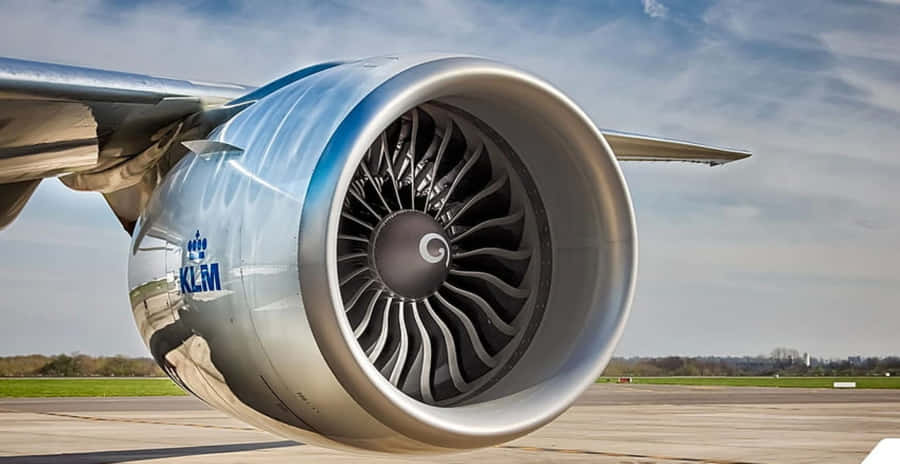This photo captures a large, high-bypass turbofan jet engine, prominently displayed under the right wing of a KLM airplane. The engine dominates the frame, showcasing its immense size and intricate details. The metallic gray front contrasts with the almost reflective white outer casing, which features blue "KLM" lettering. The dark fan blades inside the engine have a striking silver edge, adding to the intricate design. The engine's surroundings include an empty concrete runway in the foreground and a flat landscape in the background with patches of green grass and brownish trees. The distant horizon appears hazy, with a mix of clouds and subtle blue sky, indicating a daytime, outdoor setting at an airport.